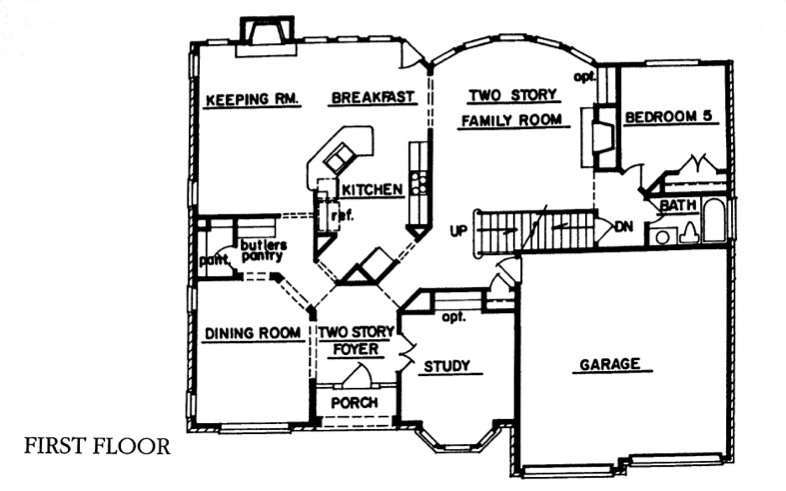This image is a top-down, black-and-white sketch of a building's first floor layout, meticulously outlining different rooms and areas without any detailed furniture representations. The labeled areas include a kitchen, study, dining room, porch, garage, pantry, bedroom, bath, and a two-story family room. 

Starting from the bottom of the image, there's a porch spanning the entire width. To the bottom left, outside the structure of the house, the label "first floor" is prominently displayed. Adjacent to the porch on the left side, the dining room is situated, which leads into the pantry toward the middle of the sketch, connecting it to the centrally located kitchen. The kitchen is one of the more detailed areas, with visible counters and walls.

On the bottom right, one of the largest labeled areas is the garage, represented by a simple black box. Directly to the left of the garage is the study. Moving to the top of the sketch, the top right corner houses a bedroom, and next to it is a bath. In the middle of the sketch, a spacious two-story family room is highlighted. On the top left corner, there's a designated breakfast area, situated just above the kitchen and to the left of the family room.

In summary, this sketch is a detailed yet simplified representation of the first floor, providing a clear layout of the main living spaces, their connections, and relative locations within the building.